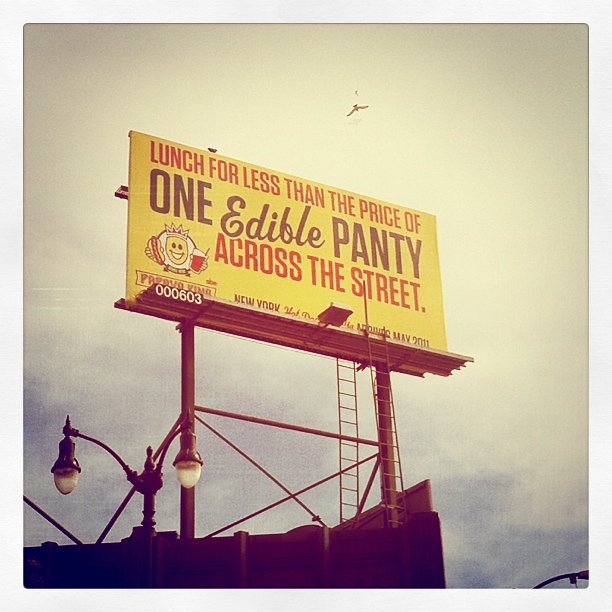A vibrant and humorous billboard is prominently displayed against a light gray and white sky, towering high above the street. The billboard is painted a bright yellow, instantly catching the eye. In bold red and brown lettering, it cheekily announces, "Lunch for less than the price of one edible panty across the street." To the left of the text, a cartoon figure with a round head, adorned with a crown, holds a hot dog in one hand and a drink in the other, adding a playful touch to the advertisement. The mischievous expression on the character’s face complements the billboard's quirky message, making it an unforgettable sight for anyone passing by.